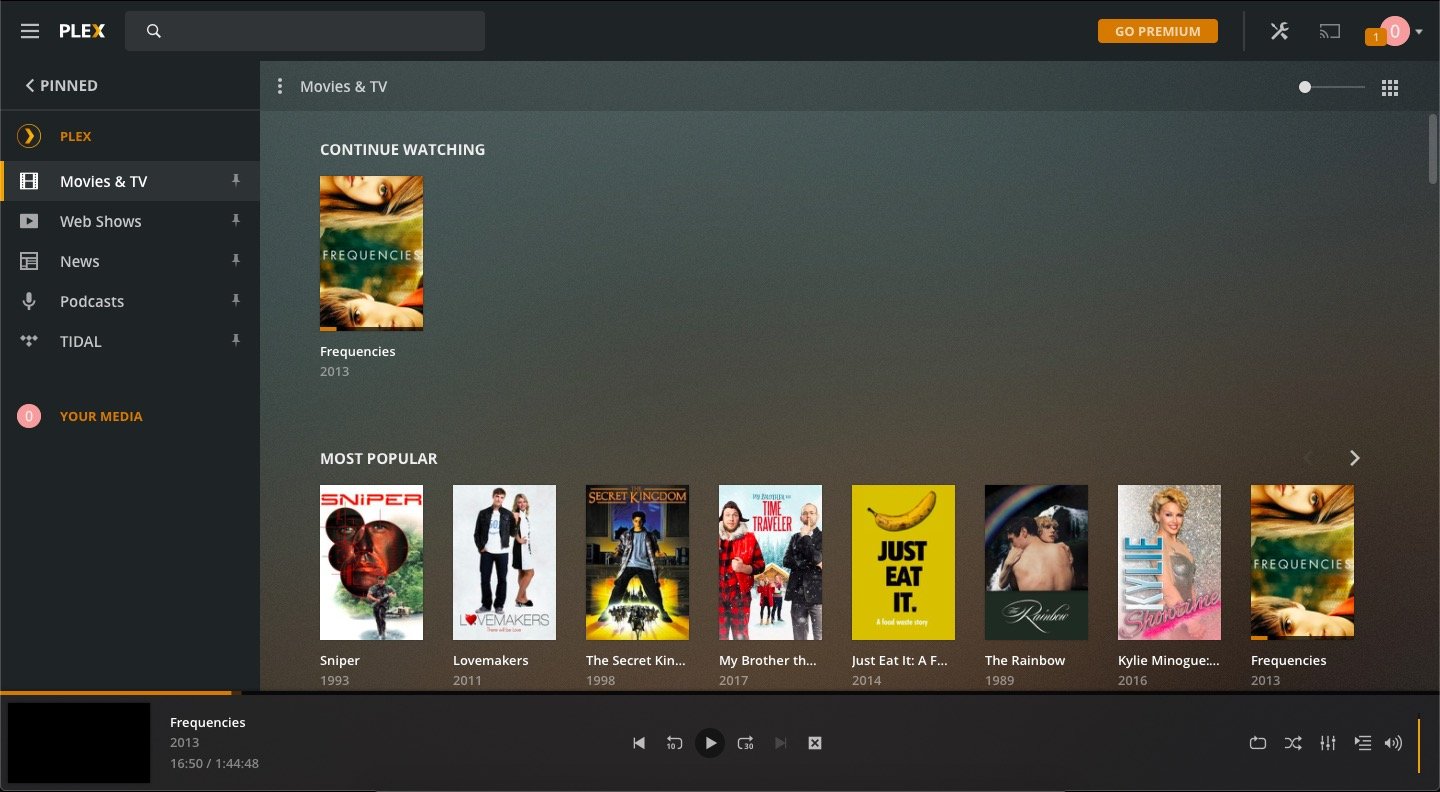The screenshot depicts a web browser featuring the Plex media server interface, highlighting various functionalities and navigable sections. 

At the top, the Plex logo is situated on the far left, followed by a search bar to its right, leaving ample space before the remaining icons on the far right. These include an orange "Go Premium" button, a settings icon, a Chromecast icon, and a profile icon marked with an orange notification badge.

The interface is divided into two main sections. On the left, a sidebar titled "Pinned" is shown, containing two subsections: "Plex" and "Your Media." Under the "Plex" subsection, there is a list comprising categories such as "Movies & TV," "Web Shows," "News," "Podcasts," and "TIDAL." The "Movies & TV" category is currently highlighted.

On the right pane, detailed content under the "Movies & TV" section is displayed. The first section here is "Continue Watching," which includes a movie titled "Frequencies" from 2013. Below that, the "Most Popular" section showcases a variety of films with their posters and respective release years, listed as follows:
- "Sniper" (1993)
- "Love Makers" (2011)
- "The Secret Kingdom" (1998)
- "My Brother the Time Traveler" (2017)
- "Just Eat It: A Food Waste Story" (2014)
- "The Rainbow" (1989)
- "Kylie Minogue: Showtime" (2016)
- "Frequencies" (2013) (listed again)

An arrow icon above the movie poster for "Frequencies" indicates more content available to the right.

The browser footer features a mini-player with "Frequencies" (2013) currently playing. On the bottom left, a small window displays the movie with its duration information. Central footer controls include a play button, a rewind 10 seconds button, a forward 30 seconds button, and an 'X' to close the player. On the far right of the footer, navigation icons such as replay, sound mixing, and volume control are located.